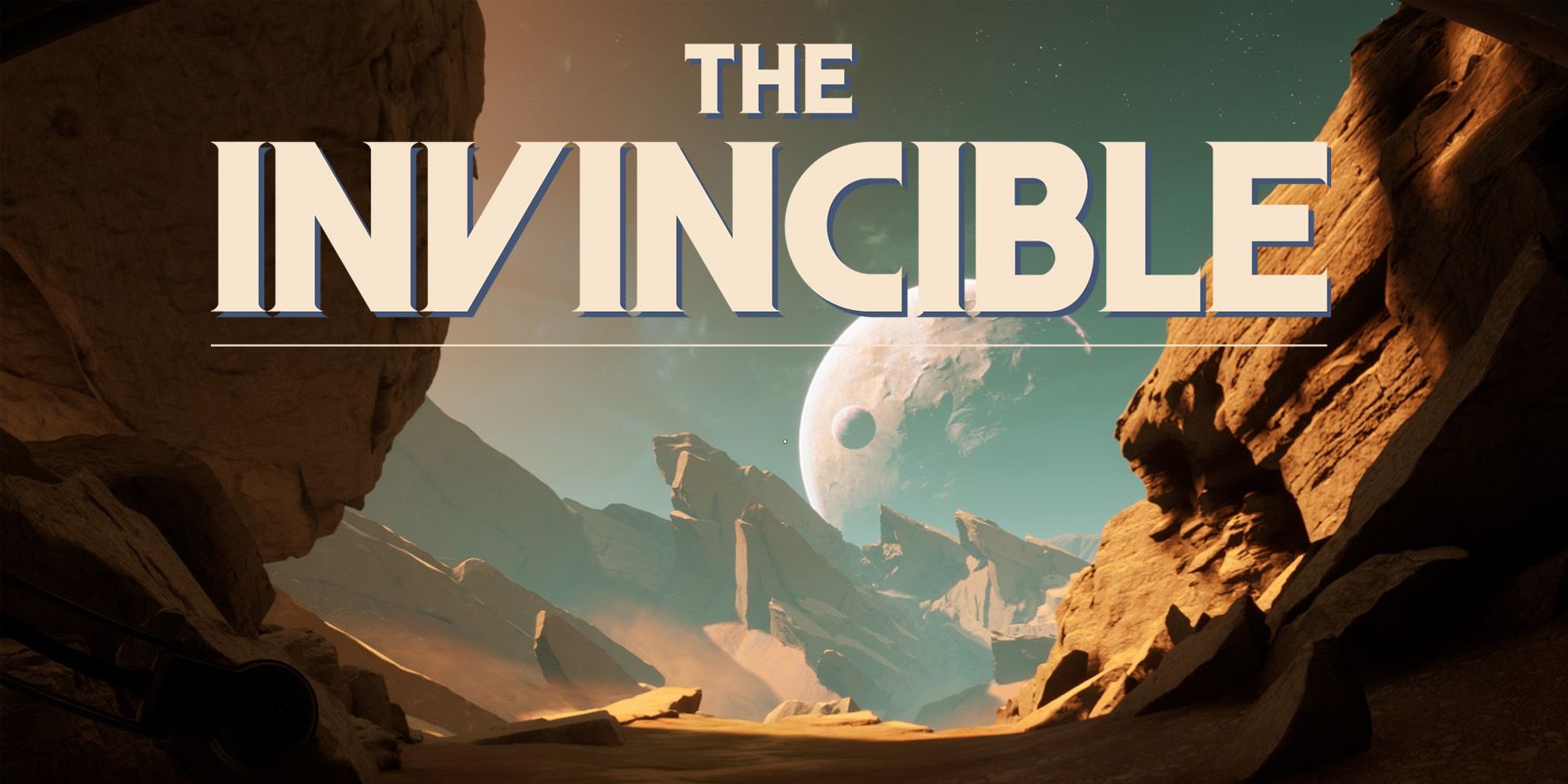The image is a detailed, rectangular drawing that is wider than it is tall, featuring a dramatic science fiction landscape. It depicts a desert-like setting with a sandy or earthen floor. Dominating the scene are imposing rocky cliffs, with brown, red, and clay hues, that edge the right and left sides of the image. In the background, sharp, tall outcroppings of rock rise from the desert floor, contributing to the otherworldly feel. The sky above is a blend of blue, pink, and purple tones, adding a surreal atmosphere to the scene. Hanging low in the sky is a large, faded planet or moon, almost transparent in its depiction. In the center of the image, prominently displayed in large white letters, are the words "The Invincible." The word "The" is small and positioned at the top, while "Invincible" is much larger and underlined in white, with the "V" slanted for emphasis. Shadows in the foreground give the impression of looking out from a cave, adding depth and contrast to the brightly lit rocky mountains outside. The intricate details and striking composition suggest that this is an illustration for a movie, TV show, or book cover.